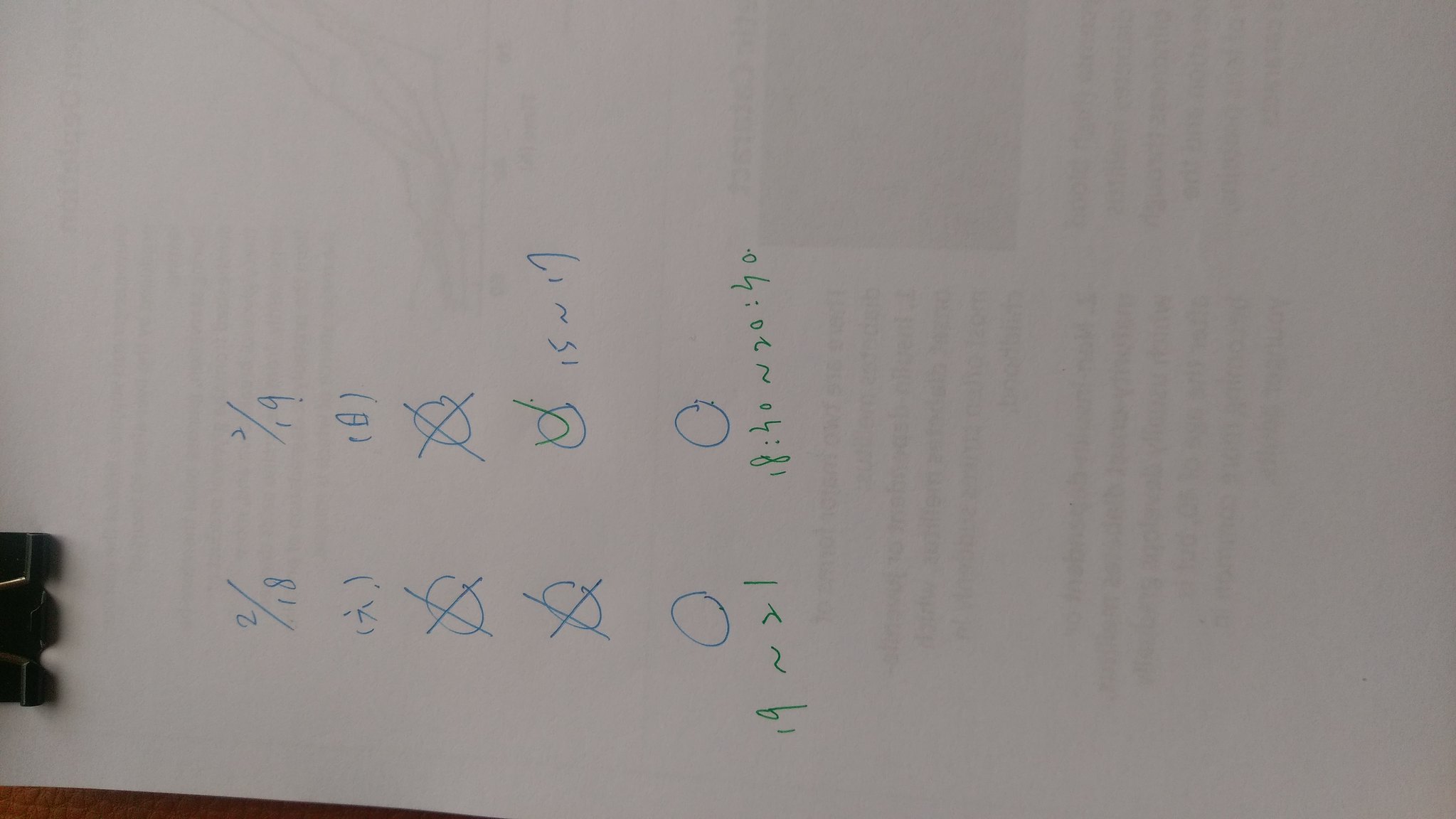This image depicts a piece of white paper with various numerical notations and symbols, drawn in a somewhat erratic, sideways manner. The paper appears to have an underlying print on the reverse side, suggesting it was flipped over to reuse. Secured at the top by a paper clamp, the sheet rests on a wooden desk. 

On the left side of the paper, the notation "2/18" is written, while "2/19" is penned on the right. Below these fractions, a scratched number that looks like "18.1" or "17.1" is visible, though the handwriting is somewhat unclear. On the right side next to it, the sequence "1 8 1" is jotted down.

There are also two zeros marked with X's through them. Another zero bears an X, and yet another zero features a U-shaped green mark, possibly meant to represent a check mark. The paper also shows the number "15" followed by an ambiguous symbol and the number "17". Below, two circles are drawn alongside the notation "19 = 21".

On the far right, a circle contains the sequence "18...30", followed by another set of symbols difficult to decipher but seemingly reading "20...30". The precise details and some of the symbols are hard to make out, contributing to the overall impression of hasty or rough sketching.